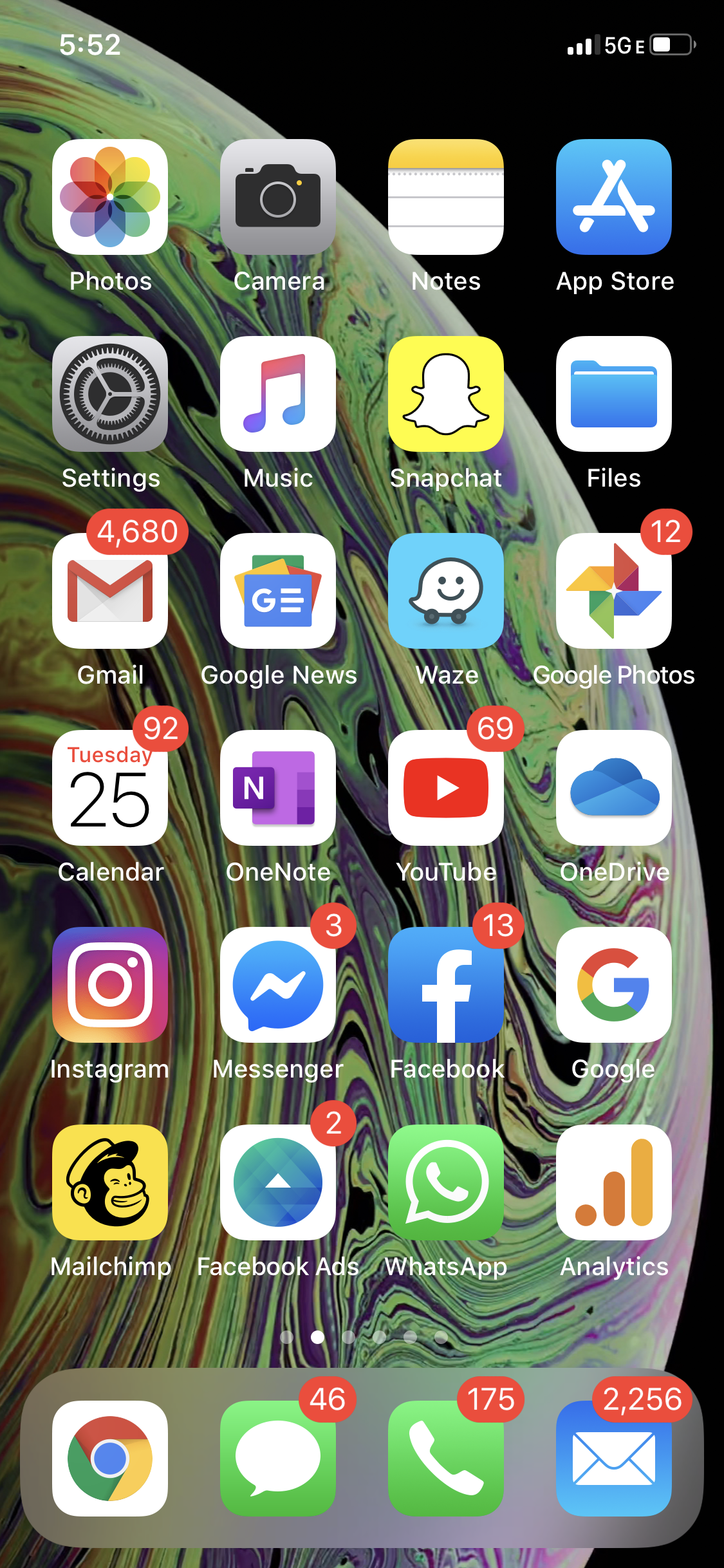A screenshot of a smartphone home screen captures a colorful and dynamic display. The background image depicts an otherworldly landscape with captivating purple, green, and white swirls, evoking the feel of an alien planet. On the home screen, various applications are neatly arranged, including Gmail, Photos, YouTube, OneDrive, Google Photos, Google News, Instagram, Messenger, Facebook, WhatsApp, Analytics, MailChimp, Files, App Store, Notes, Camera, and Settings.

Prominently displayed at the top is the Gmail app, revealing an overwhelming 2,256 unread emails. Similarly daunting, the phone's inbox features 175 missed calls and 46 unread messages. Another Gmail icon, located at the bottom, indicates an even more staggering total of 4,680 unread emails. The navigation app, Waze, is shown as well, hinting at the user's affinity for keeping various utilities at their fingertips. The image overall curates the essence of a busy and connected digital life.